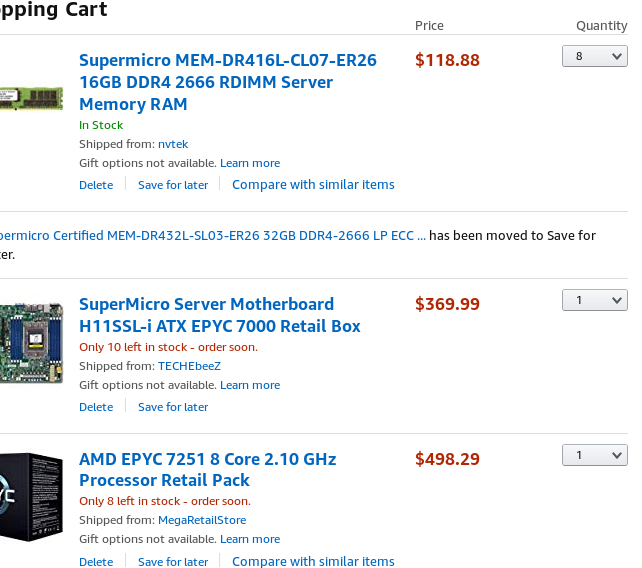This screenshot from Amazon is slightly cut off on the left edge. In the top-left corner, “shopping cart” is partially visible. Below, the first item listed is "Super Micro MEM-DR416L-CL07-ER26, 16 GB DDR4-2666 RDIMM Server Memory RAM," priced at $118.88. It’s indicated to be in stock and shipped from NVTEK, with gift options not available. Options to delete, save for later, or compare similar items are provided, and the quantity is set to 8. 

The next item has been moved to "Save for Later" and is a "Super Micro Server Motherboard H11SSL-I ATX EPYC 7000," priced at $369.99. There are only 10 units left in stock, with a note to order soon, and it’s shipped from TECHEBEEZ, with no gift options available. Options to delete or save for later are given, with a quantity of 1.

The final item is an "AMD EPYC 7251 8-Core 2.10 GHz Processor Retail Pack," priced at $498.29. There are only 8 units left in stock, with a note to order soon, and it’s shipped from Mega Retail Store, with gift options not available. Options to delete, save for later, or compare with similar items are provided, with a quantity of 1.